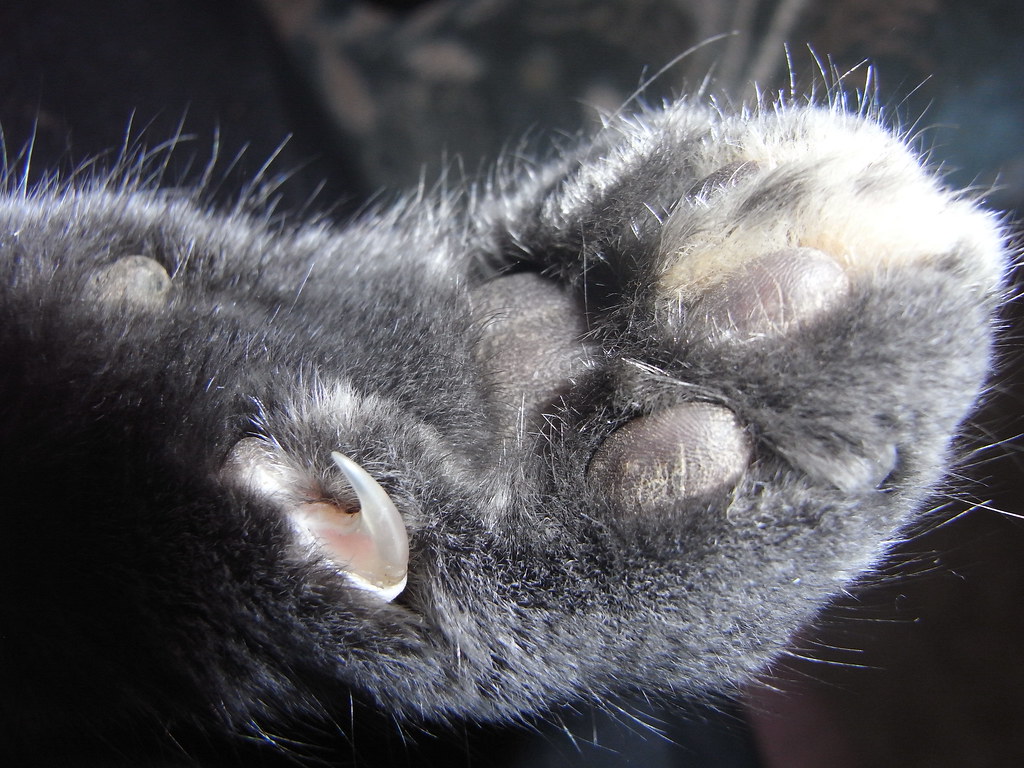This image is an extremely close-up photograph of a cat's front paw, capturing intricate details. The paw features plush, grayish-black fur with touches of white highlights where light reflects off it, suggesting a unique texture of both short and slightly longer hairs. The photo emphasizes the underside of the paw, showcasing the dark gray paw pads, known as beams. One claw on the thumb position is slightly extended, while the other claws remain retracted. The overall background is black, drawing focus entirely to the paw. The extreme zoom and side perspective reveal only a couple of the paw's toes, which appear a light purple in the light.